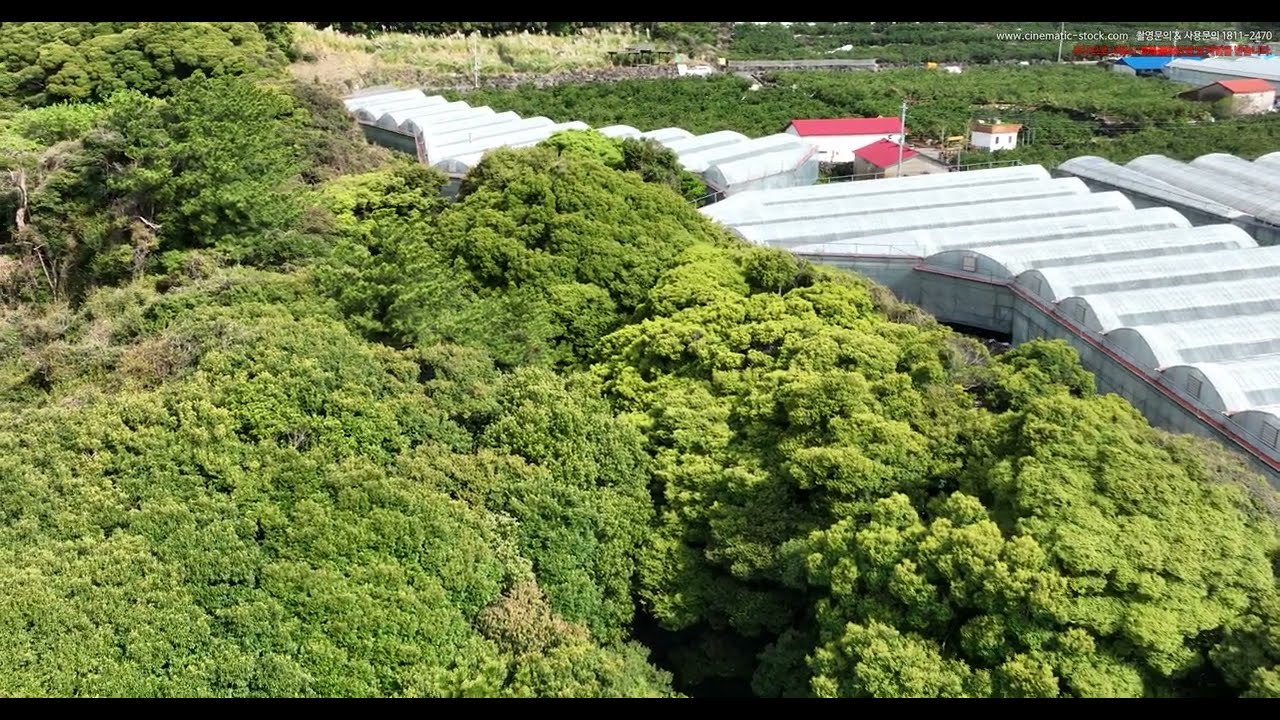The image depicts an aerial view of a series of white greenhouses arranged in an L-shaped formation that begins from the center-right and extends toward the left middle of the image. These greenhouses feature small, rounded roofs and are linearly connected at their sides but not quite joined at the top. The foreground is dominated by a dense array of tall, bushy trees with vibrant green leaves that extend diagonally from the top left to the bottom right of the image. Behind the greenhouses, additional parts of the structures are partially obscured by the large trees. In the distance, smaller white buildings with brownish-red roofs are visible, set against more areas of lush greenery and vegetation. There is text at the top of the image that reads "www.cinematicstock.com" in white letters, followed by Korean characters and the number "2470." Below that, there is additional red text that is not legible.